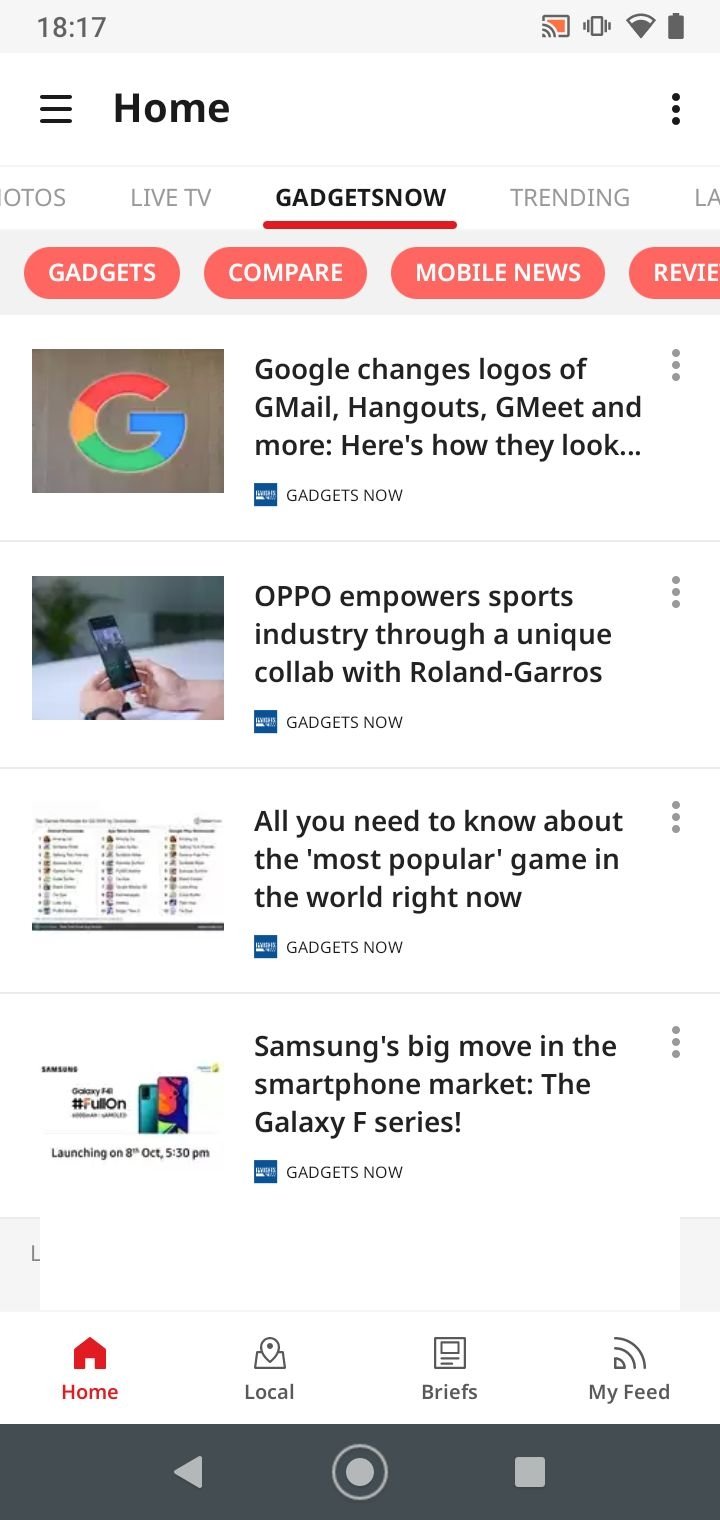Certainly! Here's a cleaned-up and detailed caption for the described image:

---

The image showcases a tablet screen with various UI elements and text. 

On the left side of the screen, the time is displayed as "8:17". Adjacent to it, a square icon is featured, which includes signal bars, vibrate, Wi-Fi, and battery indicators in the bottom left corner.

Below this section, the interface shows three horizontal lines stacked on top of each other on the left side, typically indicating a menu or navigation icon. In the center, the "Home" button is present, and on the right side, there are three vertically stacked dots, symbolizing more options or settings.

The main content area displays partially visible text cut off on the left which likely reads as "Photos". Below this, there is text indicating categories or sections such as "Live TV," "Gadgets," "Trending," and others. 

There is a red button with white font labeled "Gadgets" followed by another button labeled "Compare." Lower on the screen, text is partially visible and appears to read "Mobile news and reviews" but is cut off.

Further down, a headline states: "Google changes logo of Gmail, Hangouts, G Meets and more. Here's how they look." This is accompanied by the iconic 'G' logo featuring red, yellow, green, and blue colors. The section is titled "Gadgets Now."

Additional headlines include:
- "OPPO empowers sports industry through a unique lab with Roland-Garros."
- "All you need to know about the most popular game in the world right now."
- "Samsung's big move in the market with the Galaxy F-series."

These headlines likely point to trending tech news and updates featured on the tablet screen.

---

This detailed caption captures the essence and specifics of the screen content as described.